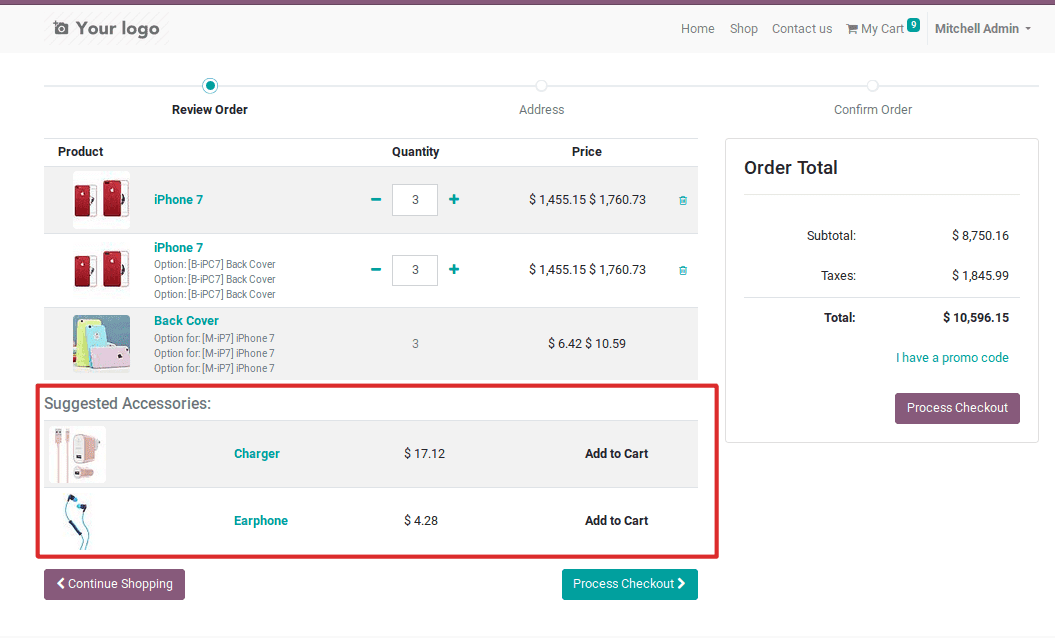A detailed caption for the image could be:

"This is a screenshot of an online store interface for ordering iPhones and iPhone accessories. At the top of the screen, placeholder text reads 'Your Logo' with a camera symbol, indicative of where users can insert their own logo. The navigation menu on the upper right corner includes options labeled 'Home,' 'Shop,' 'Contact Us,' 'My Cart,' and 'Mitchell Admin.' 

The screen is in landscape orientation, displaying the 'Review Order' stage of the ordering process, which is step one, followed by 'Address' and 'Confirm Order.' Listed products include an iPhone 7, with three units priced at $14.55.15 each and another priced at $17.60.73. Another item, also labeled iPhone 7 with various options, shows a similar quantity and pricing. The next item is a back cover with selected options, three of which are priced at $6.42 and $10.59 each respectively. 

Below the product list is a red box highlighting suggested accessories such as a charger and earphones. 

To the right, an order summary box presents the subtotal of $8,750.16, taxes amounting to $18,459, and the total cost as $10,596.15. An option to enter a promo code is available, along with a button that says 'Process Checkout.' "